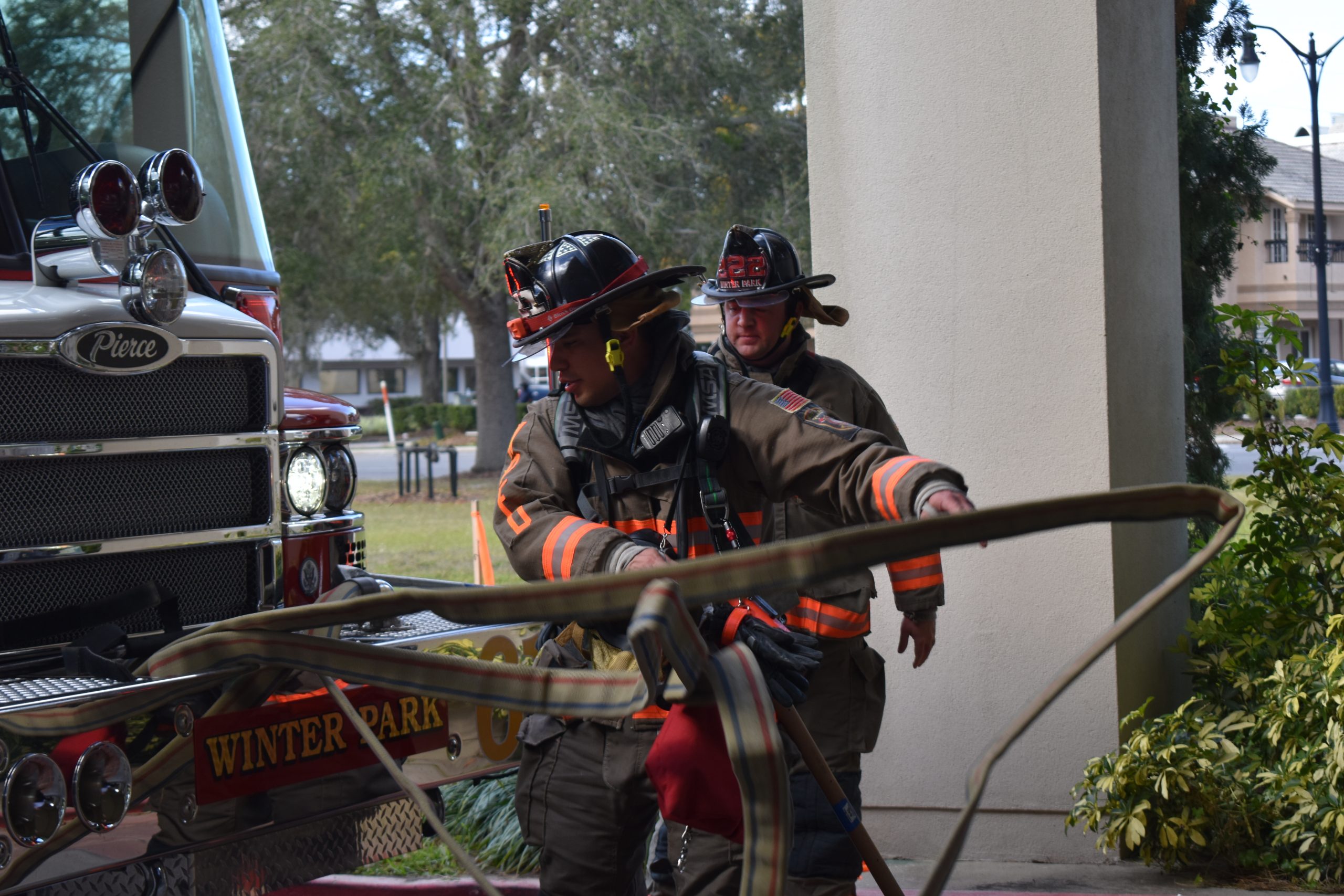In this detailed daytime photograph, two firemen are actively pulling out a flat-looking fire hose adorned with blue and red stripes from the front of a large, red Peterbilt fire truck. The truck, prominently featuring the name "Winter Park" on its chrome grill, is equipped with numerous lights and a shiny chrome bumper. The firemen, dressed in dark brown coats with fluorescent orange accents and full gear including helmets, are in motion, with one in the forefront working on the hose while the other stands behind. They appear to be responding to a fire nearby.

The background showcases a well-maintained setting with lush green trees and bushes, indicating it might be spring or summer. A light tan stucco column and some low bushes frame the scene on the right, while a nice-looking apartment building is visible behind them on the left. The fire truck is positioned facing the right side of the image, and the photograph captures the sunlit setting from a straight-on standing perspective. The composition and colors suggest an organized and residential neighborhood, with various shades of green, brown, red, black, yellow, tan, beige, and off-white adding to the overall harmony of the image.